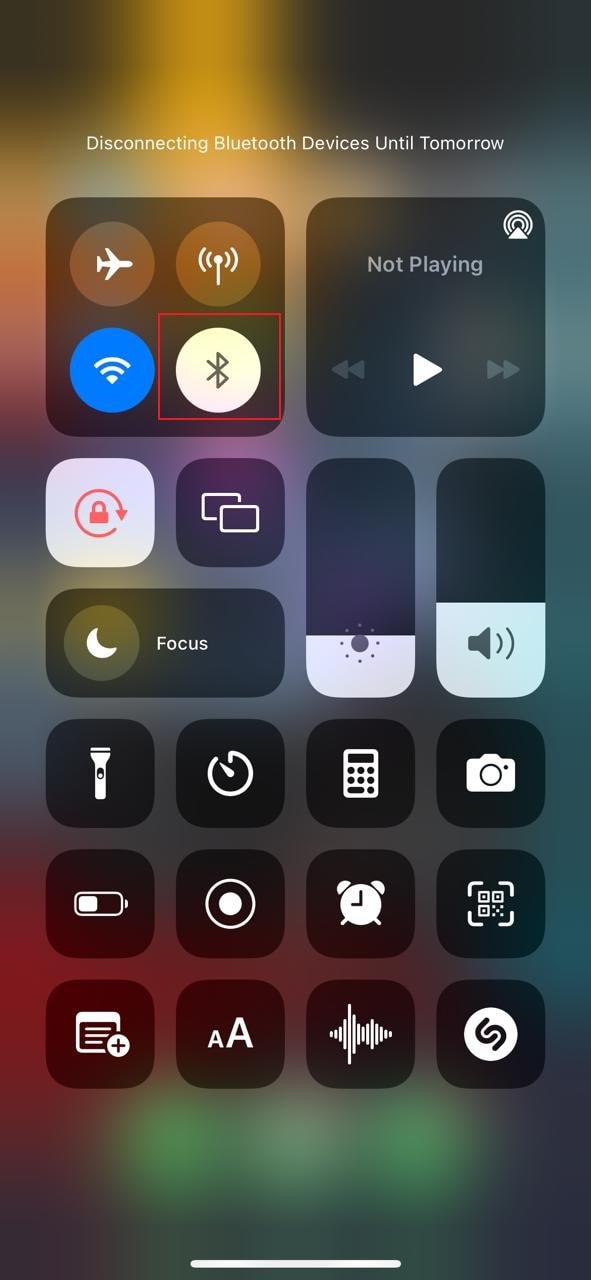This image is a screenshot from a mobile phone, showcasing a notification-rich interface. The background features a variety of color gradients and blurs: starting with the top left corner in black, transitioning into a strip of yellow extending about two inches, then reverting to black along the edges. The middle section of the screen showcases a blend of gray, blue, pink, purple, and red hues, becoming green toward the bottom, all appearing slightly blurred.

About an inch down from the top, in small white text, there's a message that reads "Disconnecting Bluetooth devices until tomorrow." Below this message, a square contains four circular icons arranged in a 2x2 grid. Adjacent to this square, on the right, a smaller square displays the text "Not playing," accompanied by playback controls, including a white play button flanked by gray rewind and fast-forward buttons.

Further down on the screen's left side, there are two squares aligned vertically, followed by a rectangle that spans about halfway across the screen. On the right side, there are two vertically aligned rectangles as well. Below these elements, a section features a row of four square icons, three stacked vertically, each with distinct symbols, all on a black background with white iconography. 

At the bottom center, flanked approximately an inch to the left and right, a white slider bar extends horizontally across the black background, completing the interface layout.